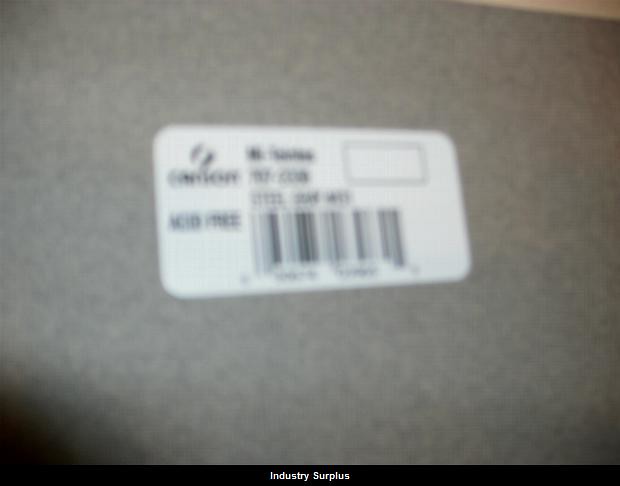This is a blurred image of what appears to be a serial code, likely for an appliance or electronic device. Although the text is difficult to read, the phrase "acid-free" is discernible, suggesting the product might be an acid-free item. The image features a barcode in the background, with several rows of numbers; while the numbers are generally unreadable, typical numerical codes are visible at the bottom. In the top left-hand corner, there seems to be the word "Canon," though it's partly obscured by an overlaid image. To the right, additional text and numbers are visible but not clearly legible. There is also a small, empty rectangular box to the side. The label itself is predominantly white on a silver background.